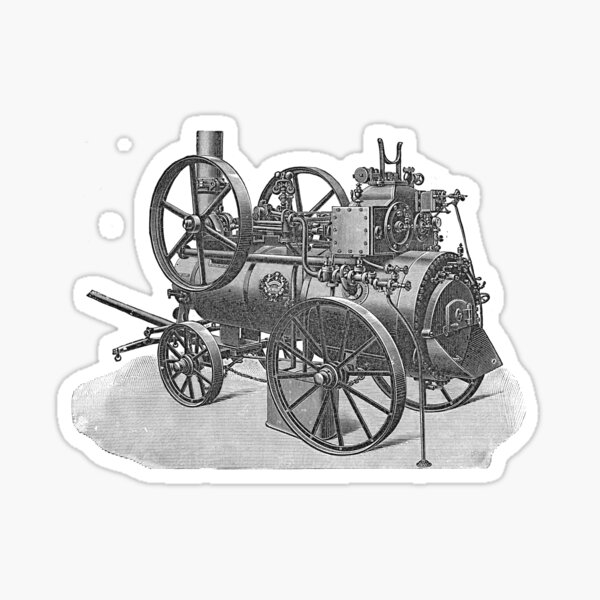This is a highly detailed, black and white illustration of an old steam engine, depicted with meticulous intricacy. The main object, centrally positioned against an eggshell-white background, has the appearance of a cut-out sticker due to its distinct white border. The artwork is reminiscent of a pencil drawing, adding to its historical charm. The engine features various sizes of wheels: two large ones at the front, smaller ones at the rear, and medium-sized wheels atop, connected by an axle. A long, robust metal tube forms the engine's base, adorned with numerous tubes, levers, spigots, handles, and dials. The front boasts a hatch for coal loading, while the rear has an exhaust pipe resembling a stove pipe. This steam-powered machine, possibly designed to be attached to a horse-drawn carriage, evokes a sense of bygone eras. The entire composition is rendered in shades of black, white, and gray, enhancing its nostalgic, vintage feel.